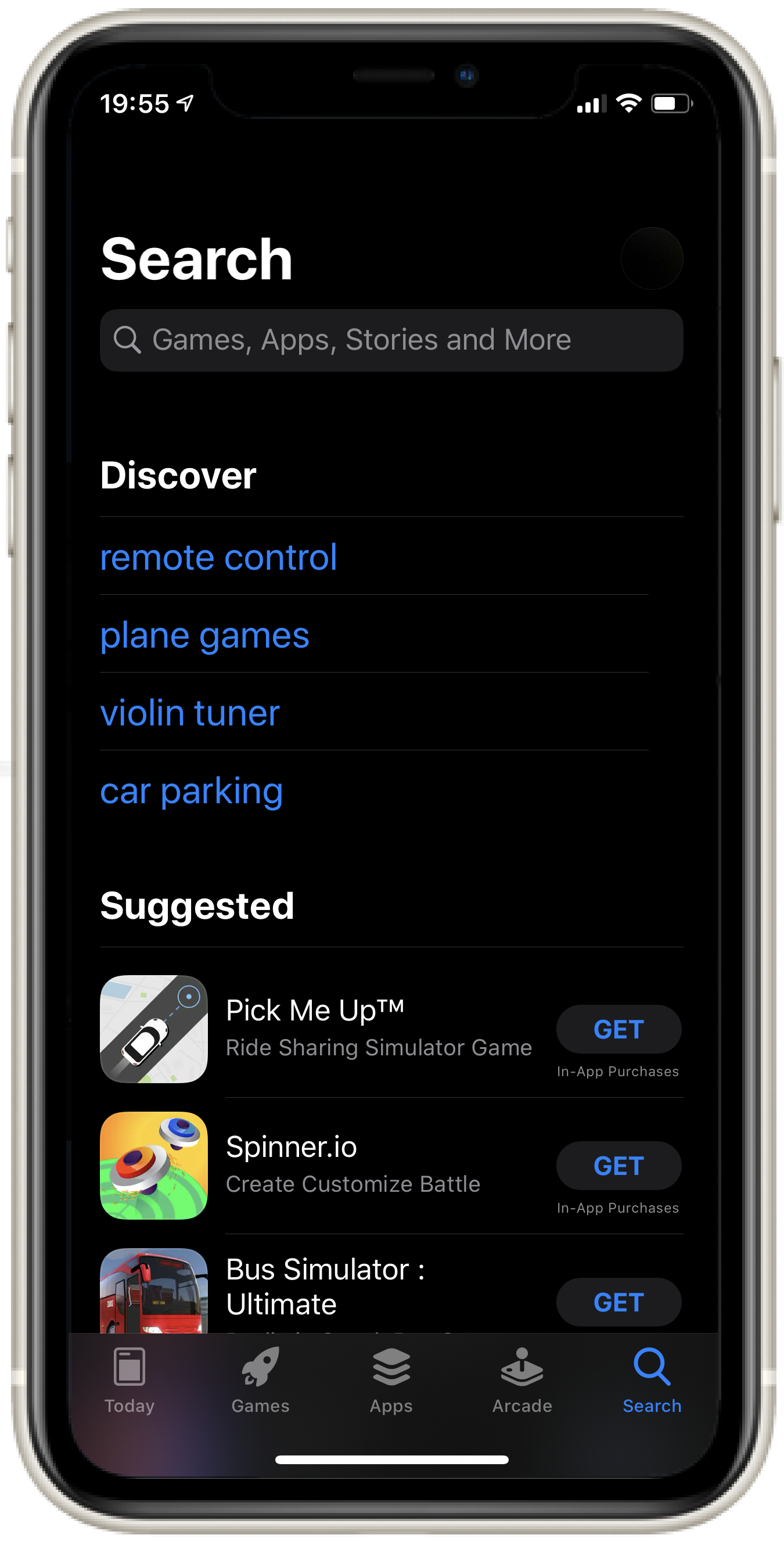This image showcases a highly detailed illustration of an iPhone, likely a mock-up rather than a real photograph, but with a very realistic appearance. The focus is on the phone itself, highlighting its physical attributes: side buttons, sleek metallic edges, and a glossy screen. 

At the top of the screen, the status bar displays the time "19:55" in the upper left-hand corner, accompanied by a paper plane icon. To the top right, next to the front-facing camera, are signal bars, a full Wi-Fi icon, and a battery indicator showing approximately 70% charge.

Below the status bar, the screen prominently features a large white text on a black background that reads "Search." Adjacent to the search field is a magnifying glass icon with the placeholder text "games, apps, stories, and more."

Further down, the screen contains text that reads "Discover" in white, followed by four lines of blue text in lowercase: "remote control," "playing games," "violin tuner," and "car parking." Underneath this section, the bold white text "Suggested" introduces a list of three apps: "Pick-Me-Up" with a "Get" button, "Spinner.io" with a "Get" button, and partially visible "Bus Simulator Ultimate" with a "Get" button.

At the bottom of the screen, a menu bar shows icons and labels for various sections: "Today" with a calendar icon, "Games" with a rocket icon, "Apps" with stacks of paper icon, "Arcade" with a joystick icon, and "Search" with a magnifying glass icon.